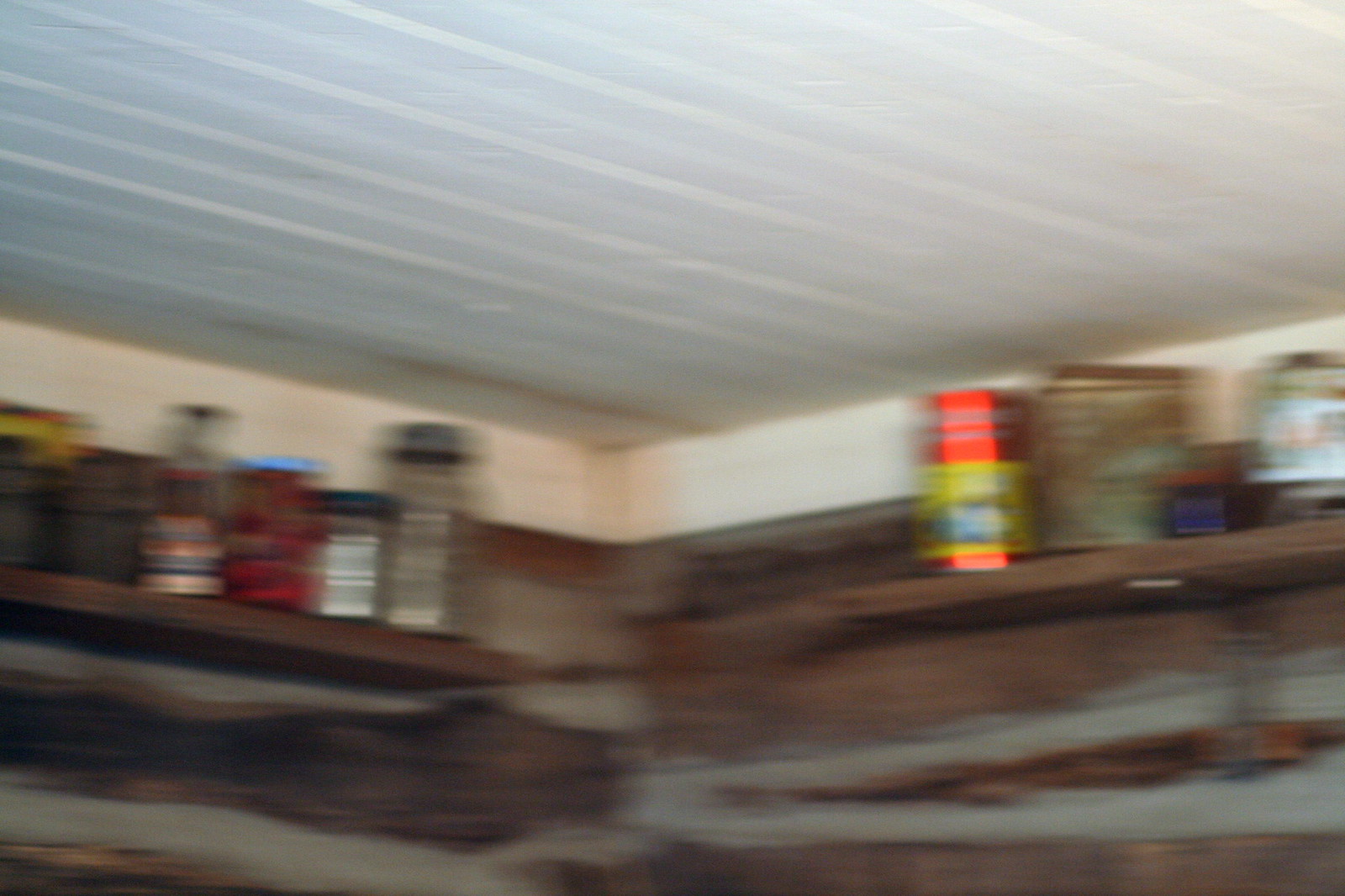This color snapshot captures a blurry image of a room with a white-painted beadboard ceiling and walls that appear to be wooden, perhaps resembling a log cabin with gray filler. The rectangular, horizontal photo prominently features the upper section of a corner where two wooden shelves meet—one on the left and one on the right, both held up by metal L-shaped brackets. Both shelves are occupied by an array of glass jars and various cylindrical containers. Notably, on the right-hand shelf, there's a container with a striking red and yellow striped label that's partly legible, along with a small blue jar nearby. The photograph is quite blurred, making it difficult to discern all the details clearly, but the arrangement of jars and containers is evident.